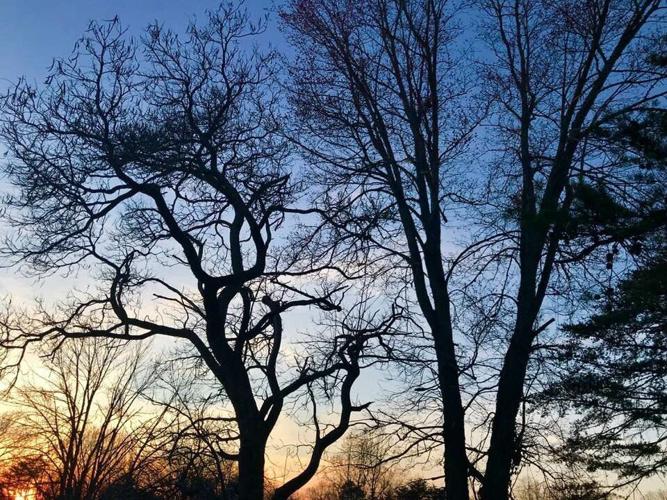In this striking image, a cluster of leafless trees stands against a vivid and gradient sky. Dominating the scene are two large trees in the foreground, one of which splits into a distinctive V shape - its stark silhouette etched against the sky. The second large tree to the left has a narrow, twisted structure with many branches. To the far right, partially visible, is a pine tree with green boughs extending into the scene. The vivid sky transitions smoothly from a deep aquamarine at the top to a lighter blue in the middle, eventually blending into a pinkish-white at the bottom. The ground beneath these towering trees is populated by shrubs and autumn-colored brown bushes, adding a layer of texture to the composition. The contrast between the bare branches and the richly hued sky creates a captivating and dynamic visual experience.